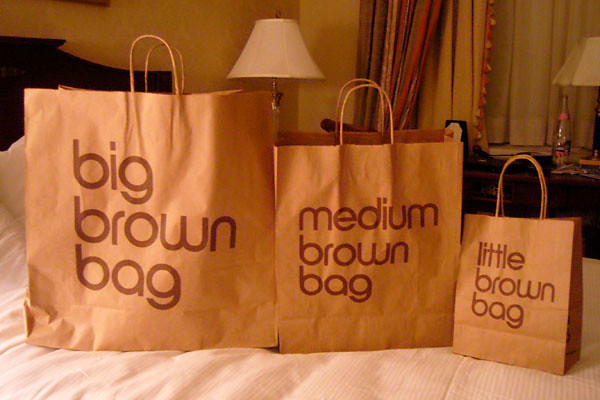In this detailed color photograph, we see three brown Bloomingdale's shopping bags of different sizes, neatly arranged in a row on a bed, creating a stair-step effect from largest to smallest. The bed, covered with a soft white comforter or quilt, is situated in what seems to be a bedroom, evidenced by the visible dark headboard and the ambient lighting from lamps, possibly on nightstands, and partially drawn curtains in the background. Each bag, crafted from brown paper with skinny handles, is clearly labeled in lowercase letters: the largest reads "big brown bag," the medium one "medium brown bag," and the smallest "little brown bag." The setting and arrangement suggest a cozy, perhaps hotel-like, environment focused mainly on the prominently displayed bags.